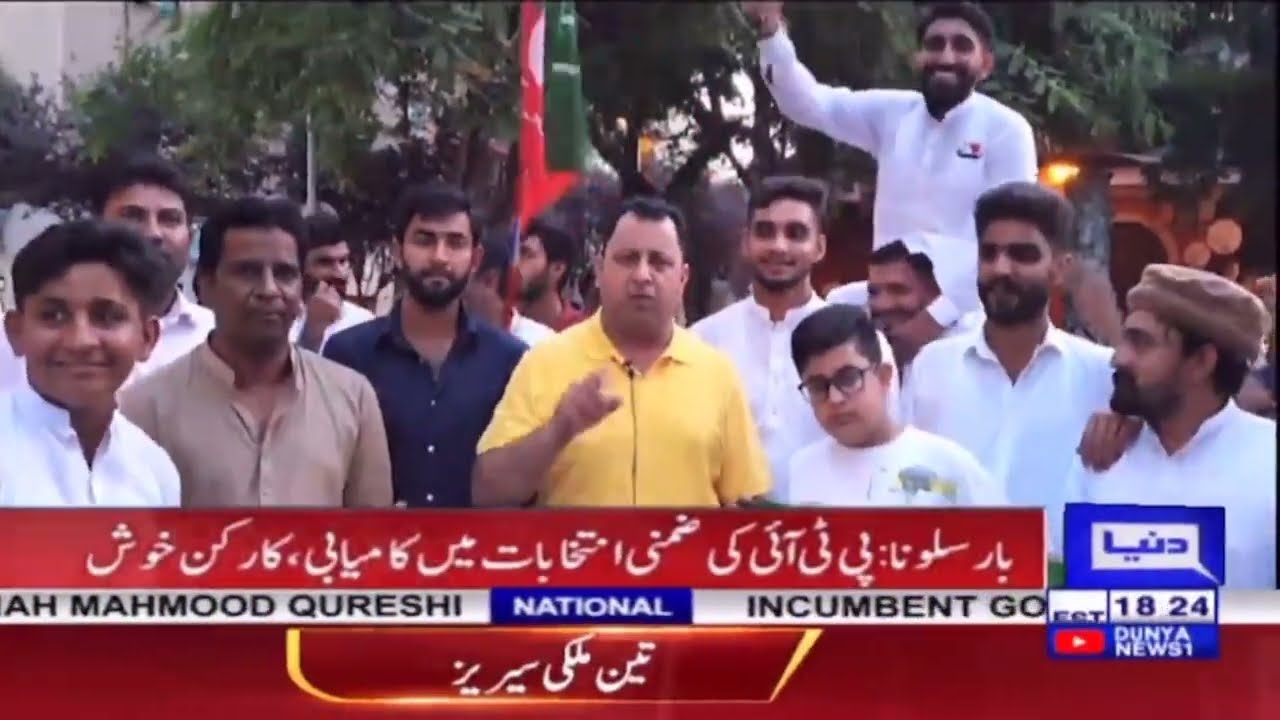The image is a detailed still shot from a television news broadcast. At the bottom of the screen, there is a large red rectangle featuring text in Arabic, typical of a news channel banner. Below this, a thinner gray strip displays scrolling English text that reads "Mahmoud Qureshi" followed by "national" in blue and "incumbent" in black. To the right, the words continue with additional English text and a small YouTube symbol. Adjacent to this is a blue rectangle with white text that says "Dunya News" along with the broadcast time.

The scene captures a group of men who are predominantly Arab-looking, with a mixture of white and colored clothing. At the center, a man in a yellow shirt with a microphone is speaking directly to the camera, pointing his finger. Surrounding him are other men; to his right stands a young man with glasses, and to the far right, a man wearing a brown cap. In the background, Indian men in white shirts are visible, with one of them lifting another man on his shoulders. This man is sporting a joyous smile with one arm raised in the air. The setting is outdoors, with trees and a building faintly discernible in the far background, indicating a political rally or public gathering.